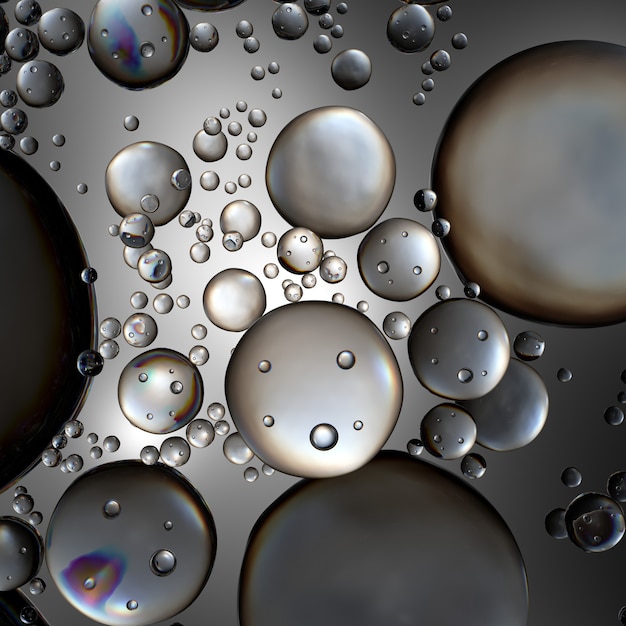The image depicts an array of bubbles of varying sizes and appearances, seemingly floating on a metallic, light gray background. The bubbles range in color and opacity, from almost clear to varying shades of gray, with some resembling water and others looking like mercury. Notably, in the left middle portion of the image, a large dark gray bubble extends off the left edge. Another significant bubble, silvery with a darker periphery, exits the frame in the upper right corner. The bottom right features a dark gray bubble partially visible as it extends off the image, above which sits a lighter gray bubble containing smaller bubbles inside it.

The upper part of the image predominantly showcases smaller and medium-sized bubbles, while two particularly large ones are positioned at the right and left edges just below the center. In the bottom region, several darker gray bubbles are present, though not as dark as the large one on the middle left. Among these, some bubbles have smaller ones on their surfaces. Intriguingly, a couple of bubbles exhibit an oily, rainbow-like reflection, adding to the image's complex visual texture. The background subtly transitions from lighter on the left and top to darker on the bottom and right, enhancing the depth and contrast of the bubble formations.